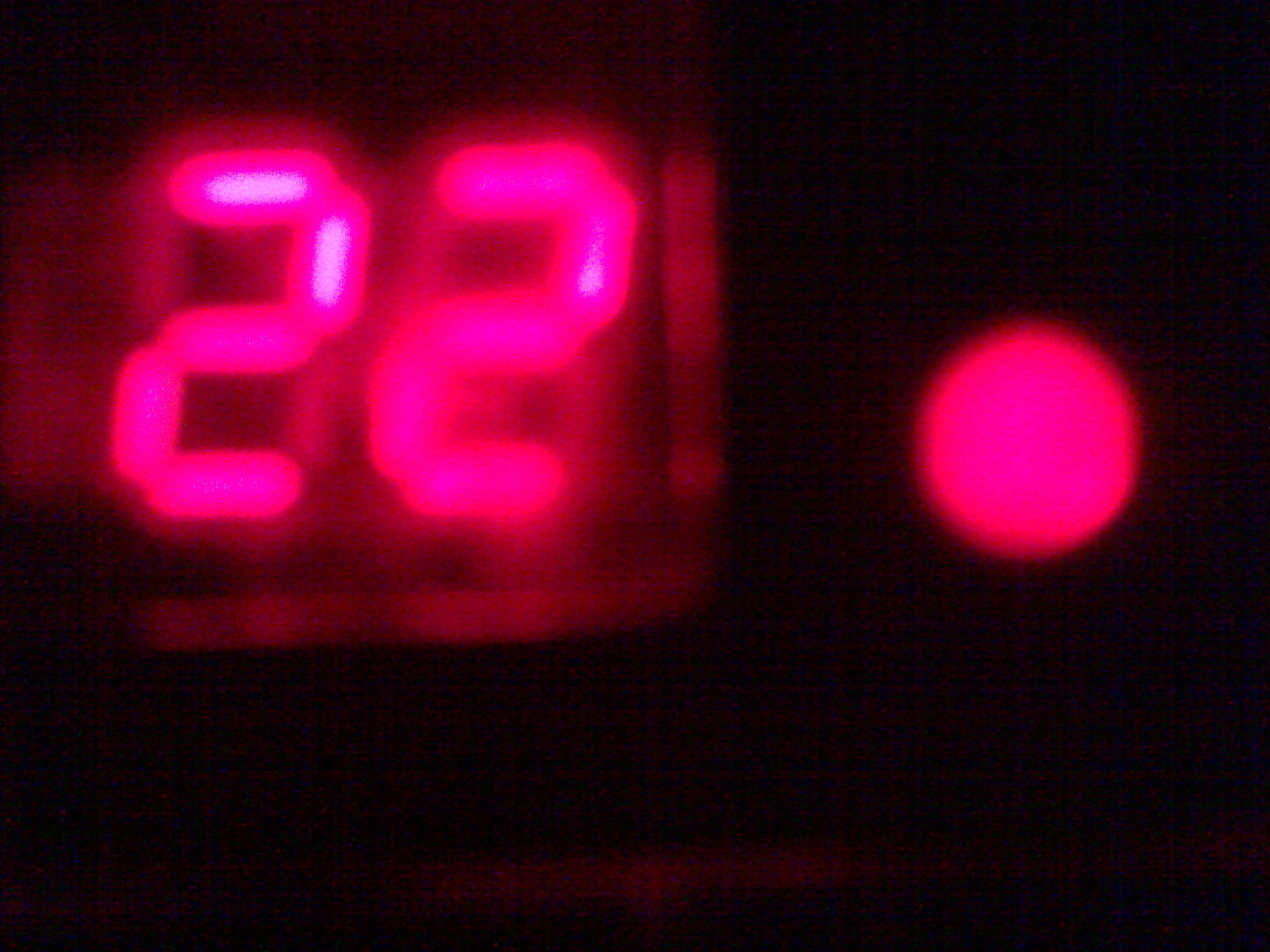The image is a blurry photograph dominated by a black background. In the upper left-hand quadrant, there is a bright hot pink neon number "22" that is lit up, occupying a bit over a quarter of the image horizontally and around half of it vertically. Just to the right of the number 22 and slightly above the middle of the right-hand side, there is a round circle also glowing in a similar hot pink color. This circle resembles a red siren light. At the bottom of the photograph, there is a faint horizontal line suggesting a surface upon which the siren may be resting. The overall dim lighting and out-of-focus quality of the image contribute to its indistinct, enigmatic appearance.